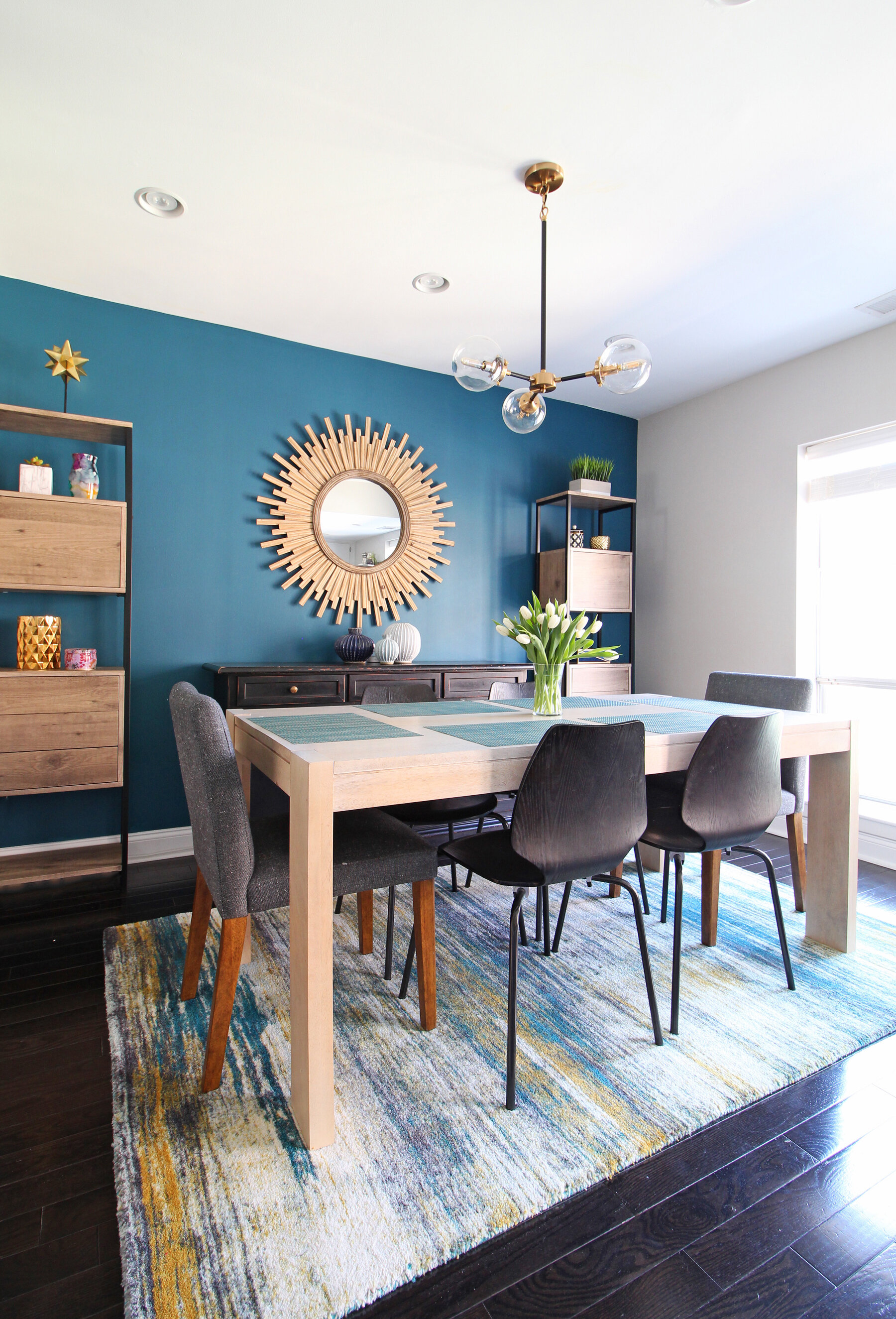The photograph depicts a modern-themed dining room corner, taken indoors during the daytime. The dining area is anchored by a dark mahogany wooden floor arranged diagonally, with a large rectangular rug featuring ombre stripes of blues, yellows, whites, and grays. Centered on the rug is a light brown, almost white, rectangular wooden dining table with squared edges, block-like legs, and a bouquet of white tulips adorning its center.

Around the table are six chairs: the two end chairs are plush, gray with cushioned backs and wooden legs, while the four side chairs are sleek black metal. To the back left, a teal-colored wall is adorned with a striking sunburst mirror above a dark brown buffet, accompanied by three vases. Flanking the buffet are tall, narrow shelving units. The right wall is painted white with a large window that streams in bright daylight, illuminating the space. Two recessed lights and a hanging light fixture with three bulbs illuminate the dining table from the white ceiling.